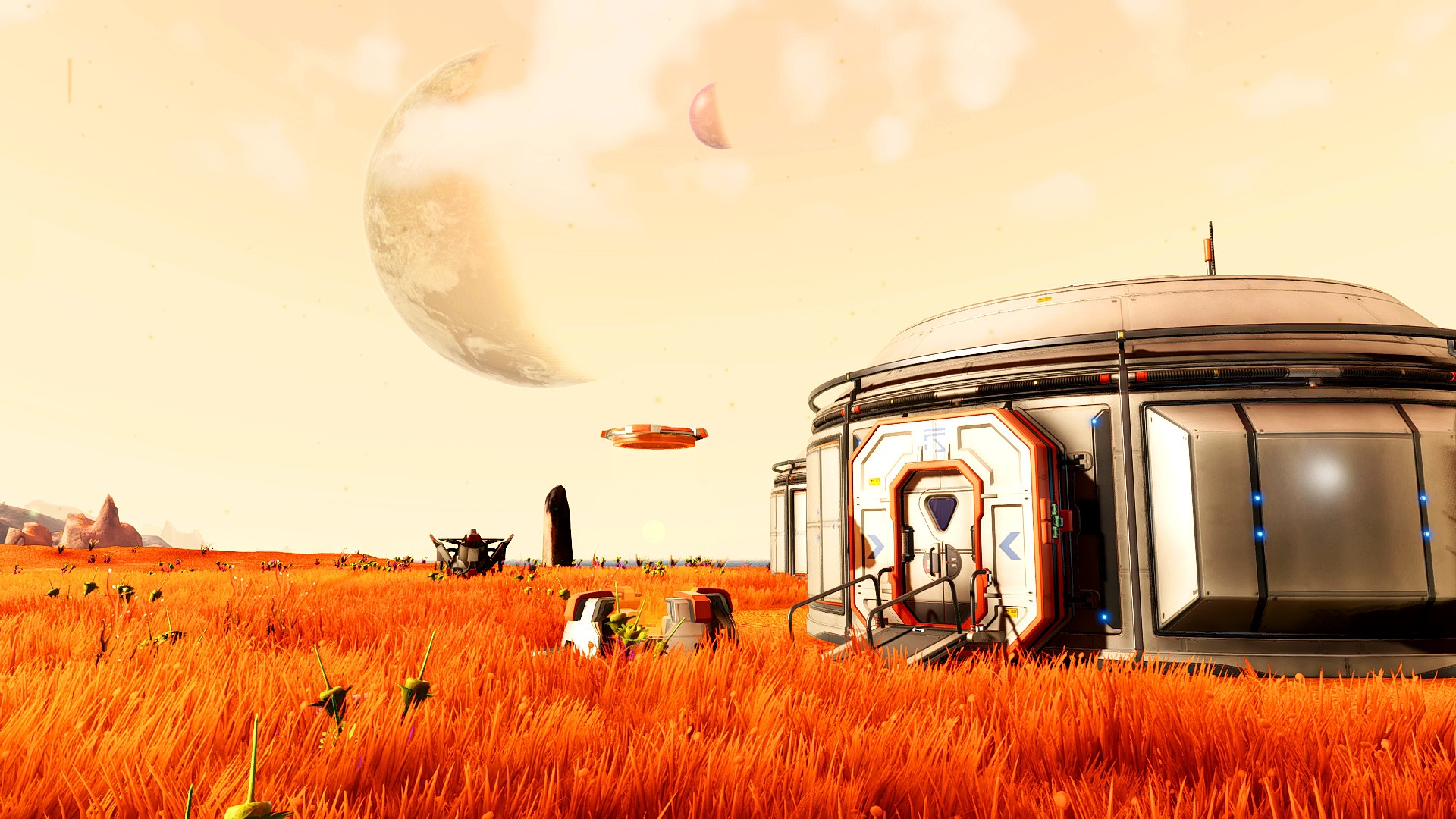This image appears to be a digitally created screenshot from a video game or other digital media, depicting an alien landscape. The ground is covered in a vibrant, pumpkin-orange grass, giving the scene an otherworldly feel. On the right side of the image stands a sleek, silver structure that resembles a futuristic habitat or hut, illuminated by glowing lights. The design of the hut is modern, characterized by a flat ramp extending from a door to the bright ground below. Dominating the upper left portion of the sky is a massive moon, partially visible and distinctly larger than Earth's moon, enhancing the extraterrestrial ambiance of the scene.